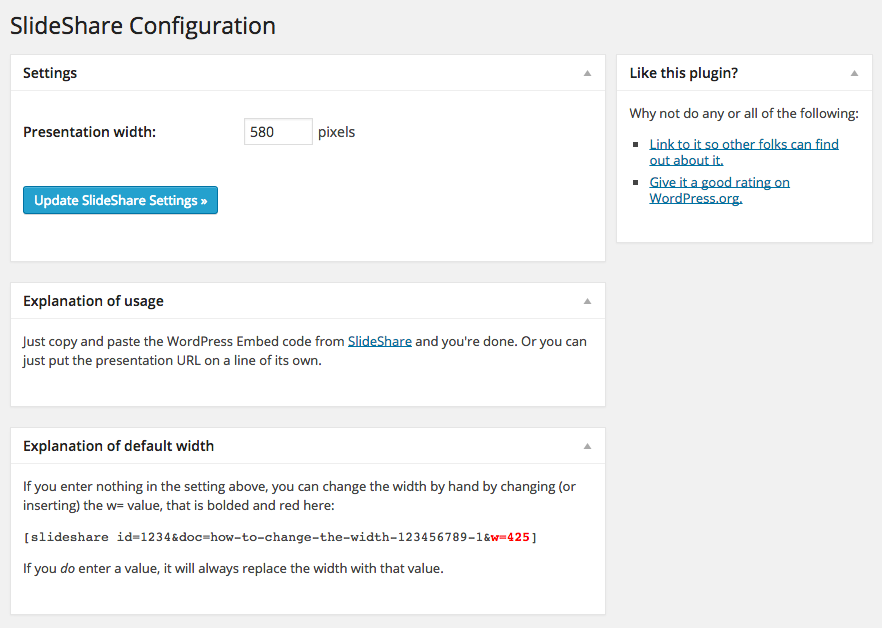**Screenshot Description: "SlideShare Configuration" Screen**

The screenshot primarily features a "SlideShare Configuration" page.

- **Header**: The top section has a gray background with bold, black text that reads "SlideShare Configuration."
  
- **Content Section**: Below the header, there are three main sections with a white background, each separated by gray lines.
  
  1. **First Block: Settings**
      - Title: "Settings" with a gray line beneath it extending from left to right and a gray arrow pointing upwards on the right side.
      - Content:
          - "Presentation Width": Labeled with a gray box next to it containing the number "580" and the unit "pixels."
          - Blue rectangular button labeled "Update SlideShare Settings" with a white asterisk adjacent to it.
          - An explanation about the usage of black lettering, indicated by a line of text reading "Explanation of Usage of Black Lettering."

  2. **Second Block: Just Copy and Paste**
      - Title: "Just Copy and Paste" followed by line of text: "the WordPress embedded code from SlideShare," with "SlideShare" underlined in blue.
      - Additional Text: Instructions on simply pasting the presentation URL on its own line.
      - Gray arrows and lines also appear to indicate sections or important elements.

  3. **Third Block: Explanation of Default Width**
      - Title: "Explanation of Default Width" with a gray line beneath and an upwards arrow on the right.
      - Content: 
          - Description of default width settings, explaining that if no width is specified, you can alter the width by changing or inserting a value with the parameter "w=" within a given code snippet.
          - Example Code: `(slideshare id=1234&doc=how-to-change-the-width-123456789-1&w=425)`
          - A note cautions that if no value is entered, a default value will replace it. The word "DO" within this note is italicized for emphasis.

- **Footer Section**: 
    - Rightmost Section: Another gray arrow points upwards with a white box asking users to "Like this plugin?" and offering links or actions users can take.
    - Actions:
        - First Bullet Point: "Link to it so other folks can find out about it," underlined and written in light blue text.
        - Second Bullet Point: "Give it a good rating on WordPress.org," emphasizing "WordPress" with capitalization.

Overall, this detailed caption provides a comprehensive breakdown of the various elements and sections within the "SlideShare Configuration" screenshot.